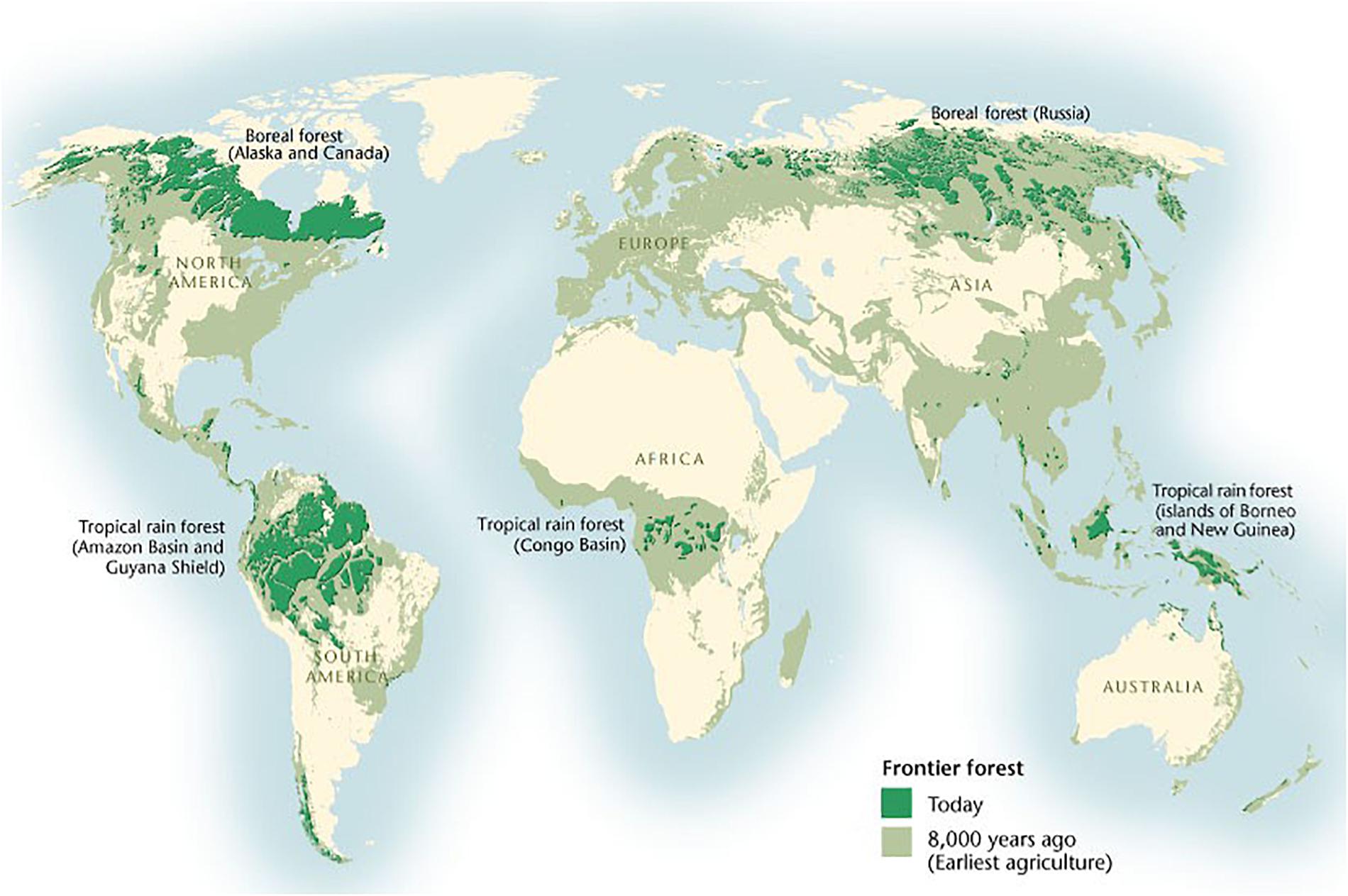This detailed image is a flat world map presented on a light blue and white background. The continents are depicted in a primarily grayish-white hue, with significant green accents indicating forest coverage. North and South America are shown on the left, while Asia, Europe, and Africa are on the right, and Australia is located at the bottom right corner, beneath India and Asia. The map is color-coded to represent "Frontier Forest" regions, using dark green to show current forest coverage and light green to illustrate forested areas from 8,000 years ago, when the earliest agriculture began.

Prominent labeled regions include the Boreal Forest in Alaska and Canada, the Tropical Rainforest in the Amazon Basin and Guyana Shield, the Tropical Rainforest in the Congo Basin, the Boreal Forest in Russia, and the Tropical Rainforest in the islands of Borneo and New Guinea. A legend situated in the bottom right corner clarifies these color distinctions: a dark green square represents the forests of today, whereas a light green square denotes areas that were forested 8,000 years ago. The map starkly illustrates how the extent of frontier forests has diminished over time, with light green areas from the past being significantly more prevalent than the dark green areas of the present.